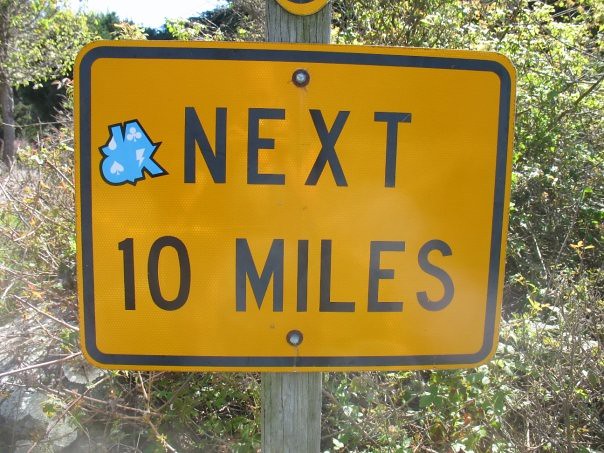In this vibrant color photograph, a bright yellow road sign is prominently displayed, securely fastened to a wooden pole that stands vertically in the center of the frame. The sign features a black border and the text "NEXT 10 MILES," indicating a cautionary message for road users. Affixed to the sign is a unique sticker in the shape of the letters "J-A-O-K." This sticker showcases a creative design in light blue, adorned with white icons of a spade, a club, and a lightning bolt, all outlined in black. The sunny day bathes the scene in ample light, causing the brush and leaves in the blurred background to appear slightly overexposed. The sign itself has light shadows and shows signs of wear, including minor cracking around the screws that attach it to the wooden pole.